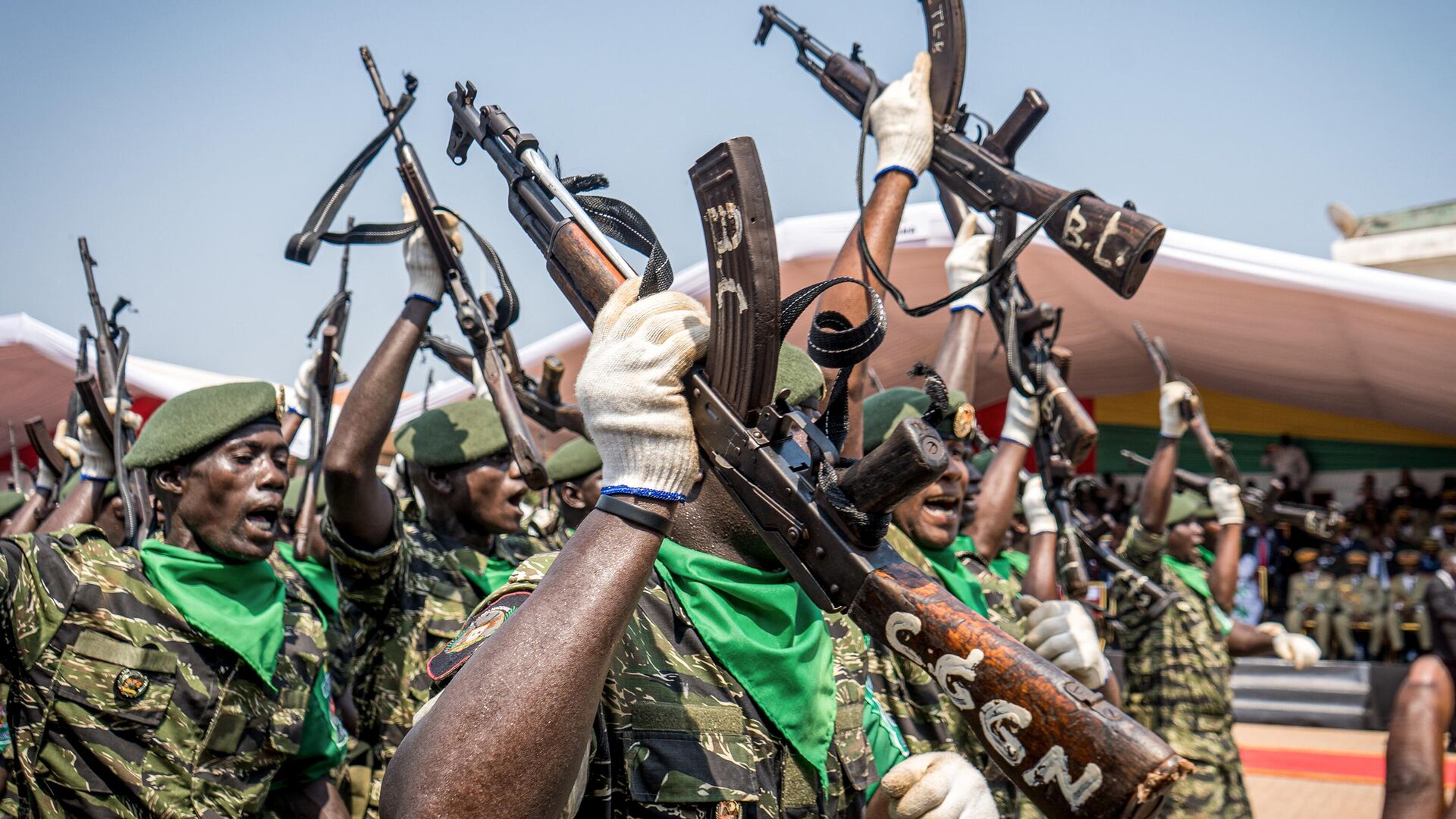This photograph depicts a group of African soldiers in a military parade. The soldiers, all with rich dark skin, are dressed in full military gear and are carrying AK-47s or similar machine guns. Each soldier's weapon bears some form of symbolic writing, although the exact details are not fully legible. The soldiers, all wearing gloves, march in unison, likely for a ceremonial purpose or to boost morale. In the background, there is a white-covered tent adorned with yellow, red, and green colors on its walls, possibly representing national or military insignia. The scene also suggests the presence of country leaders and possibly other spectators, illustrating a significant national or military event.